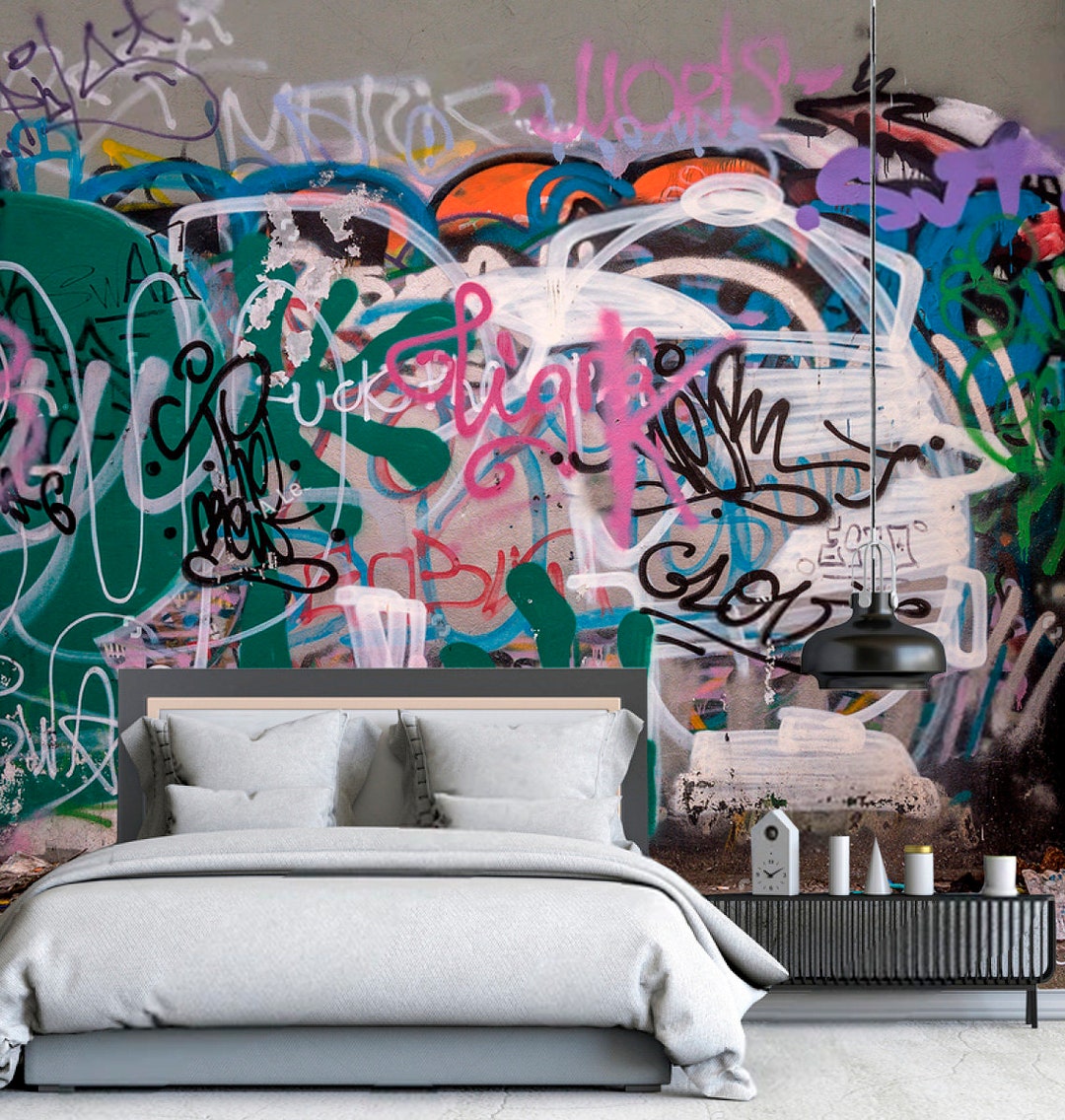This image captures a bedroom dominated by an intriguing juxtaposition of modern comfort and urban flair. The room features a cozy, neatly made bed, likely a queen size, with a rectangular gray headboard and footboard. The bed is adorned with a soft gray comforter and white pillows, creating a plush, inviting appearance. Adjacent to the bed on the right side is an upcycled, silver side table characterized by its textured lines. The table is relatively long for a bedside piece and holds five white objects: two white candles, a pillar candle, a cone candle, and a clock shaped like a house.

However, the most striking element of the room is the wall behind the bed, which appears as a cement canvas covered in dynamic graffiti. The graffiti displays an array of colors, including deep greens, light greens, pinks, purples, blues, oranges, and blacks, with scribbles, drawings, and stylized letters that are difficult to decipher. The wall is predominantly gray but showcases various layered elements, such as a prominent big white area that seems painted over with other colors, and a notable pink 'K' in the middle. The left side of the wall features a significant amount of green, transitioning to mostly blacks and whites on the right. From the top right corner of the image, a long cord or wire descends to a cylindrical black light fixture positioned above the side table. This eclectic mix of street art-inspired chaos and serene, modern design creates a captivating contrast within the room.